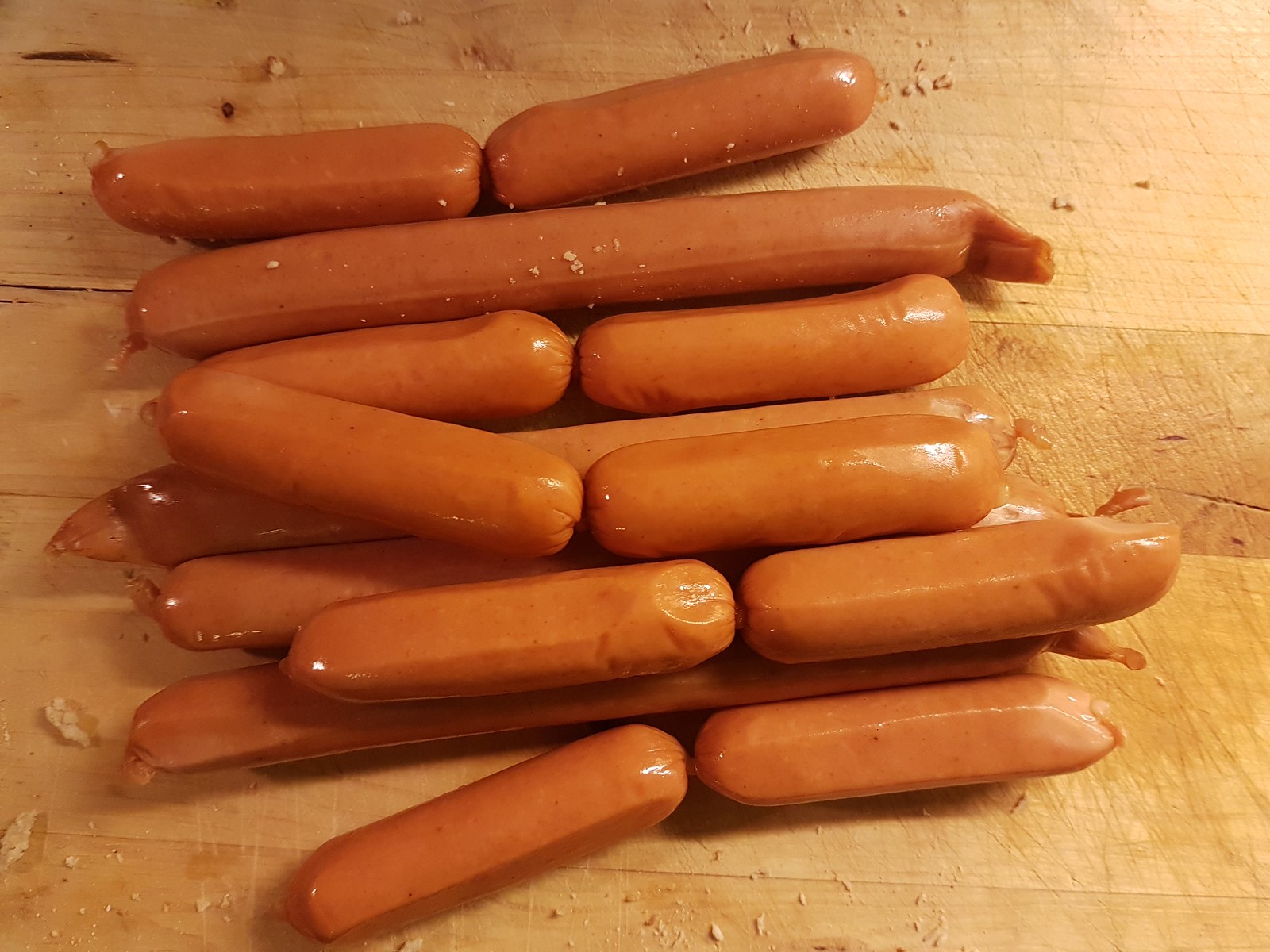This detailed photograph showcases a collection of hot dogs laid out on a light tan, unfinished wooden surface that appears to be a cutting board. The cutting board features natural marks, including chips, indentations, and scuffs likely left by knife cuts from previous use. Scattered around the cutting board and atop several of the hot dogs are light tan breadcrumbs, suggesting that bread may have been sliced on it previously.

The focal point of the image is a pile of around 15 to 20 hot dogs of varying lengths. The majority of these hot dogs are mini-sized, often linked in pairs, while a few are full-length, likely double the size of the mini ones. These hot dogs all share a consistent cooked appearance with a reddish-pink color. The specific arrangement and details, including the breadcrumb dusting and the variations in hot dog sizes and linking, add texture and context to the photograph, emphasizing the simple yet detailed scene.